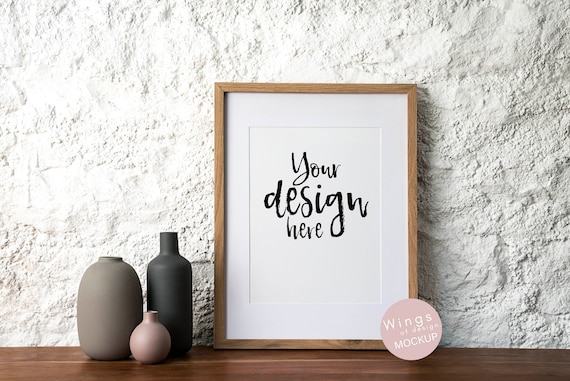The image displays a photorealistic digital mock-up set against a white, textured, stucco or concrete wall. Central to the composition is a wooden-framed, vertical rectangular sign with a light brown border. The sign features white cursive text reading "Your Design Here" on a slightly off-white background. Positioned in the bottom right corner of the frame is a pink round sticker with the white text "Wings of Design Mock-Up."

Beneath the sign, there's a dark brown wooden shelf supporting three decorative clay vases of varying shapes. From left to right, the first vase is a cylindrical light gray bottle, the center vase resembles a vertical shampoo bottle, and the last one is a rounded vase akin to a small perfume bottle with a push button on top.